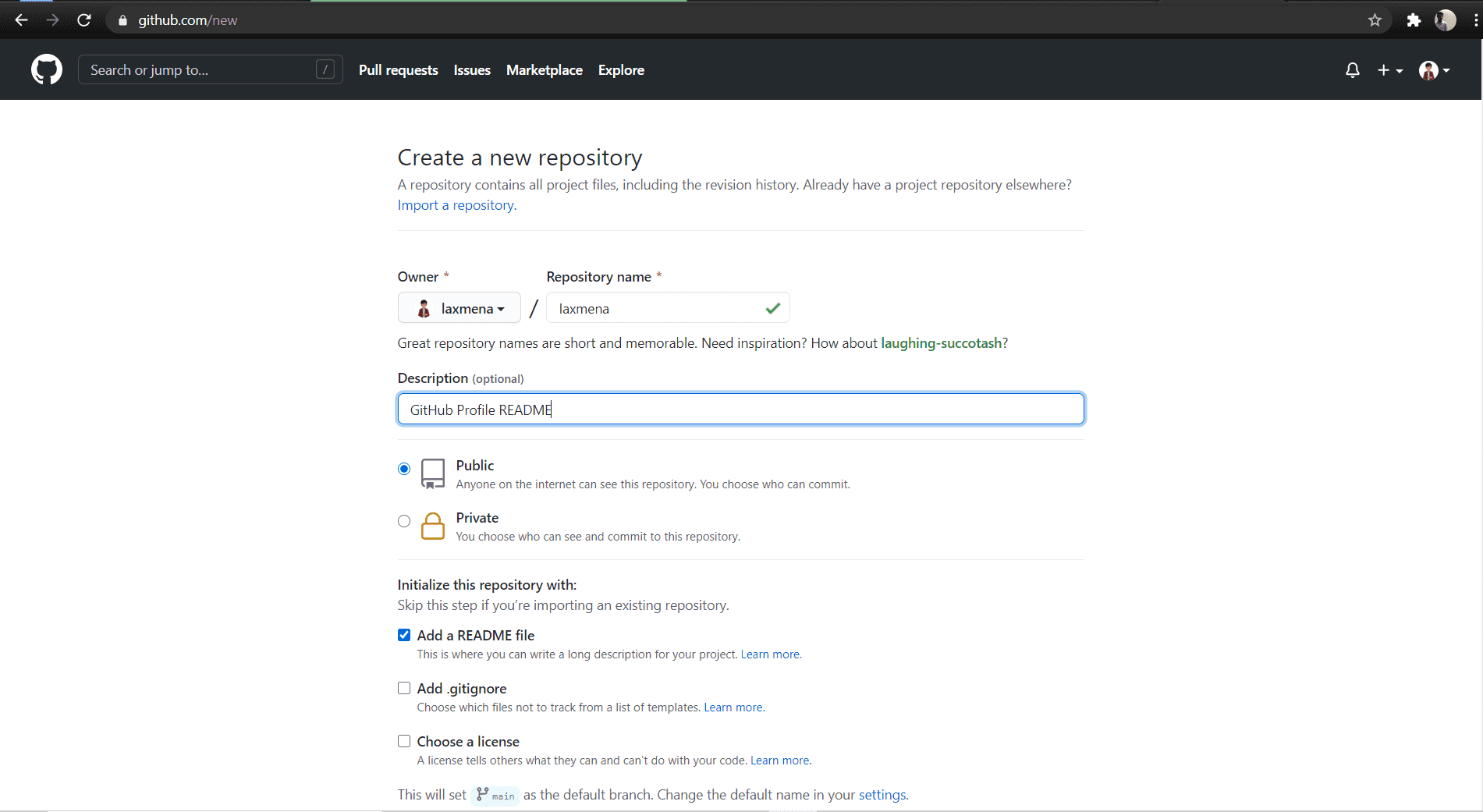At the top of the image is a black navigation bar featuring a white arrow pointing left and a gray arrow pointing right. Directly adjacent is a white circular refresh icon, followed by a gray bar displaying a locked padlock icon and the URL "github.com/how." To the right of the URL, a series of icons are present: a star, a puzzle piece, a circle containing a person, and a vertical stack of three equally sized and shaped dots. On the left side of this bar, the white silhouette of the GitHub cat logo is visible, with the text "Search or jump to" next to it. Further right, there are tabs labeled "Pull Requests," "Issues," "Marketplace," and "Explore." Additional icons to the right include a bell, a plus sign, a minus sign, another circle with a person inside, and a dash.

The main content of the page has a white background and features the heading "Create a new repository." The description below explains that a repository contains all project files, including the revision history. There is an inviting link in blue, "Import a repository," for those who already have a project elsewhere. Following this section, fields for "Owner" and "Repository name" are marked with asterisks indicating required input. A text box below shows the entry "laxmina/laxmina," accompanied by a green checkmark. Additional information suggests, "Great repository names are short and memorable. Need inspiration? How about laughing-secatash?"